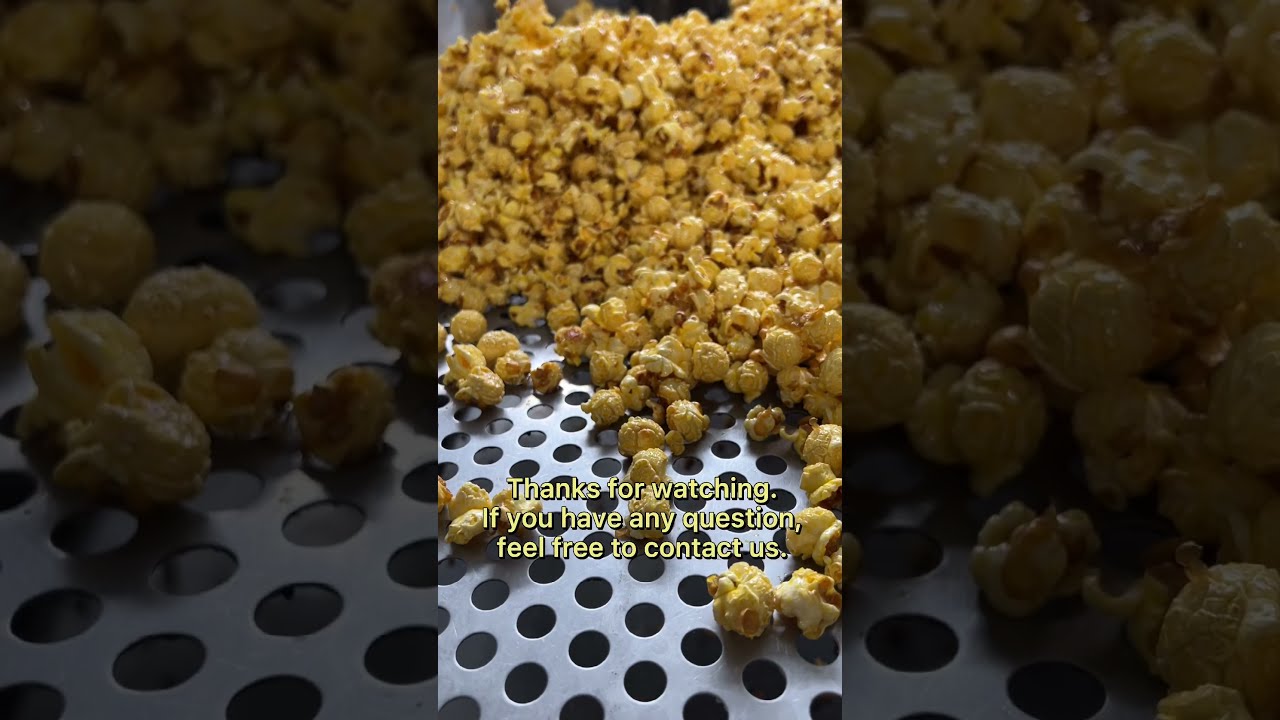The image features a large pile of caramel-colored popcorn or kettle corn, filling most of the frame. The popcorn has a shiny, sugary coating, indicative of kettle corn, and varies in size and fluffiness. The background appears to be a black surface with white overlay featuring holes, allowing the dark background to peek through. Across the top of the image, in yellow font, there's a caption stating, "Thanks for watching. If you have any questions, feel free to contact us." Despite the informative text, the central focus remains on the popcorn, which seems to be the main subject of the image.